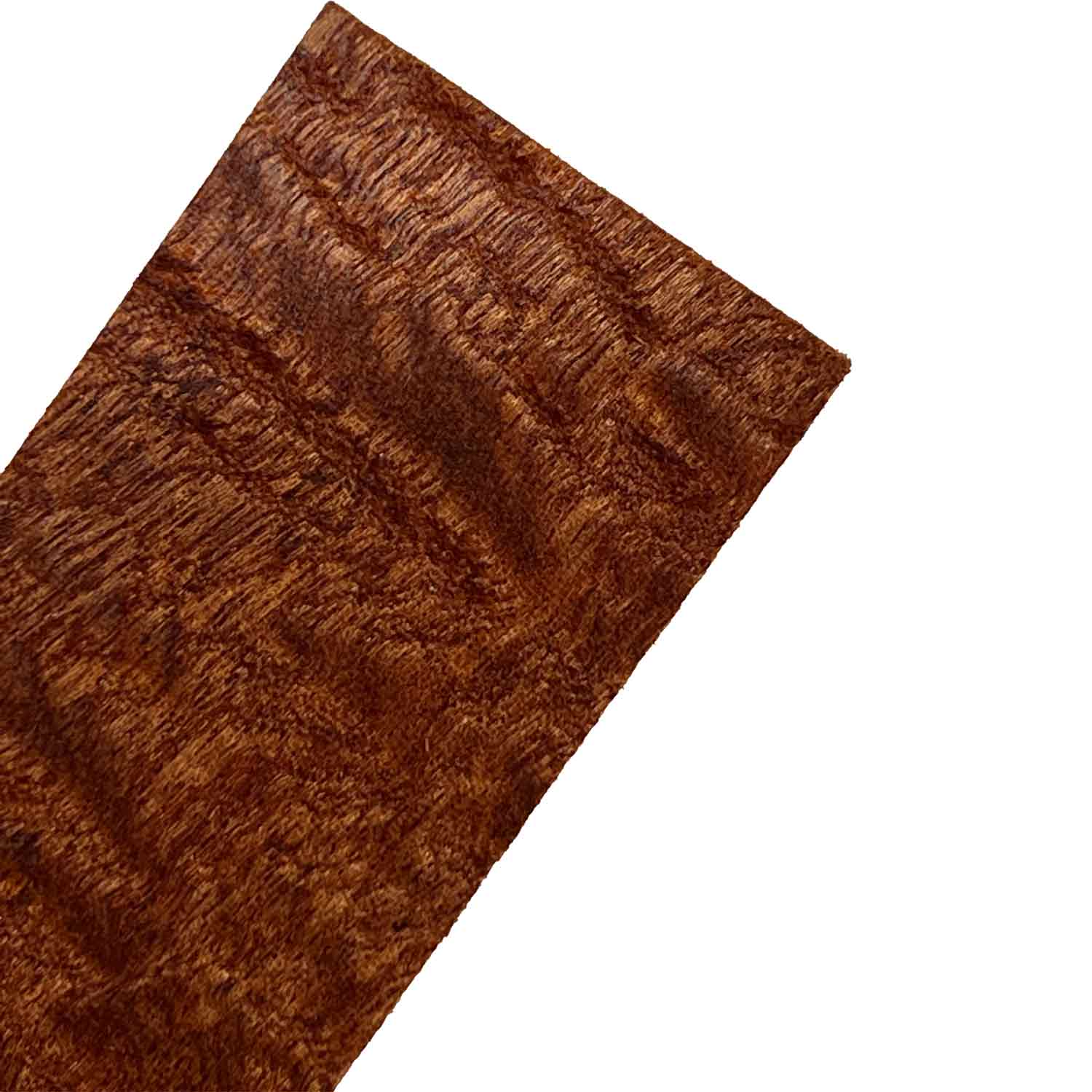The image features a centrally positioned piece of brown cloth, potentially silk due to its subtle shine. It predominantly showcases shades of brown, hinting at a bronze or mahogany chestnut hue, with light creating a shimmering effect that introduces hints of gold. The cloth displays indistinct designs and folds, especially towards the left-hand side, where it is folded in two places, contributing a geometric pattern to its almost rectangular shape. The background is plain white, emphasizing the single object's presence in the image, taken by a real person, and devoid of any text.